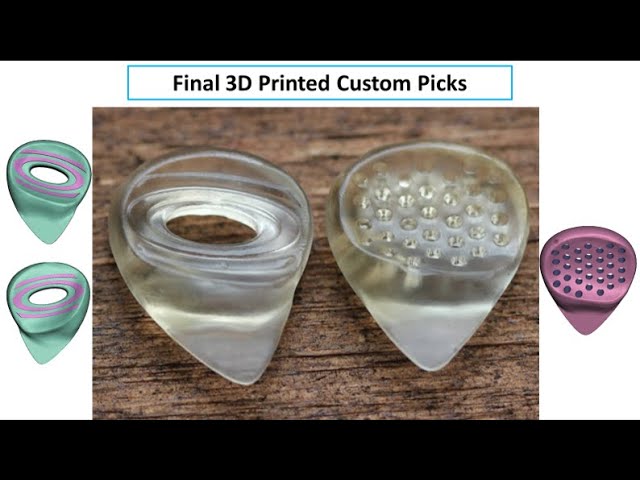This horizontally oriented image showcases an advertisement for final 3D printed custom guitar picks. It features a black bar at both the top and bottom of the image. Below the top bar, printed in black text within a blue rectangular outline, is the heading "Final 3D Printed Custom Picks."

In the center of the photo, placed on a wooden table, are two clear, translucent guitar picks. Each pick features a distinctive design: the left pick has an intricate swirl pattern, while the right pick is adorned with numerous tiny diamonds. Both picks exhibit ergonomic shapes with curved surfaces and small tabs extending from their lower edges, designed to enhance grip and playability.

To the left of these clear picks, there are two light green picks with purple swirl patterns. To the right, there's a fully purple pick, embedded with tiny purple gemstones, adding a touch of elegance and uniqueness to the collection.